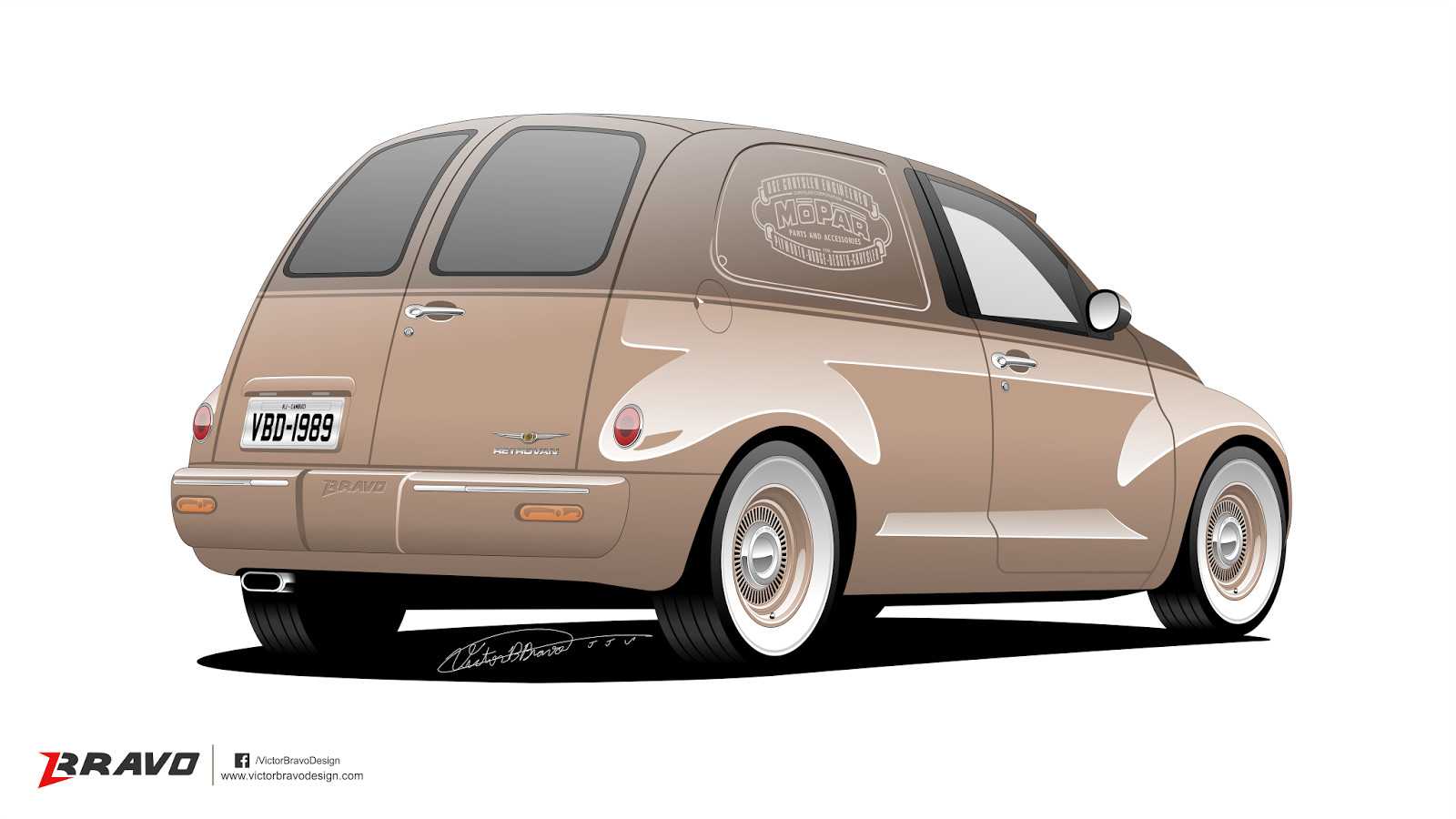This image depicts a computer-generated drawing of a car oriented towards the right. The vehicle features a two-tone color scheme with a light brown or beige bottom and a slightly darker top half. The car is detailed with white walls on the wheels and light beige hubcaps. The back window appears tinted or possibly mirrored, adding to its sleek appearance. A notable license plate reads VBD-1989 and is positioned at the back, towards the left. There is a partially visible, opaque logo on the back window on the passenger side, featuring white text that is difficult to read. The shadow beneath the car is distinctly drawn in black, and towards the rear, it incorporates a signature. In the bottom left corner of the image, the word "Bravo" is prominently displayed in stylized black lettering, adjacent to additional, less legible text. The image also includes a Facebook logo, further emphasizing its digitally crafted nature.